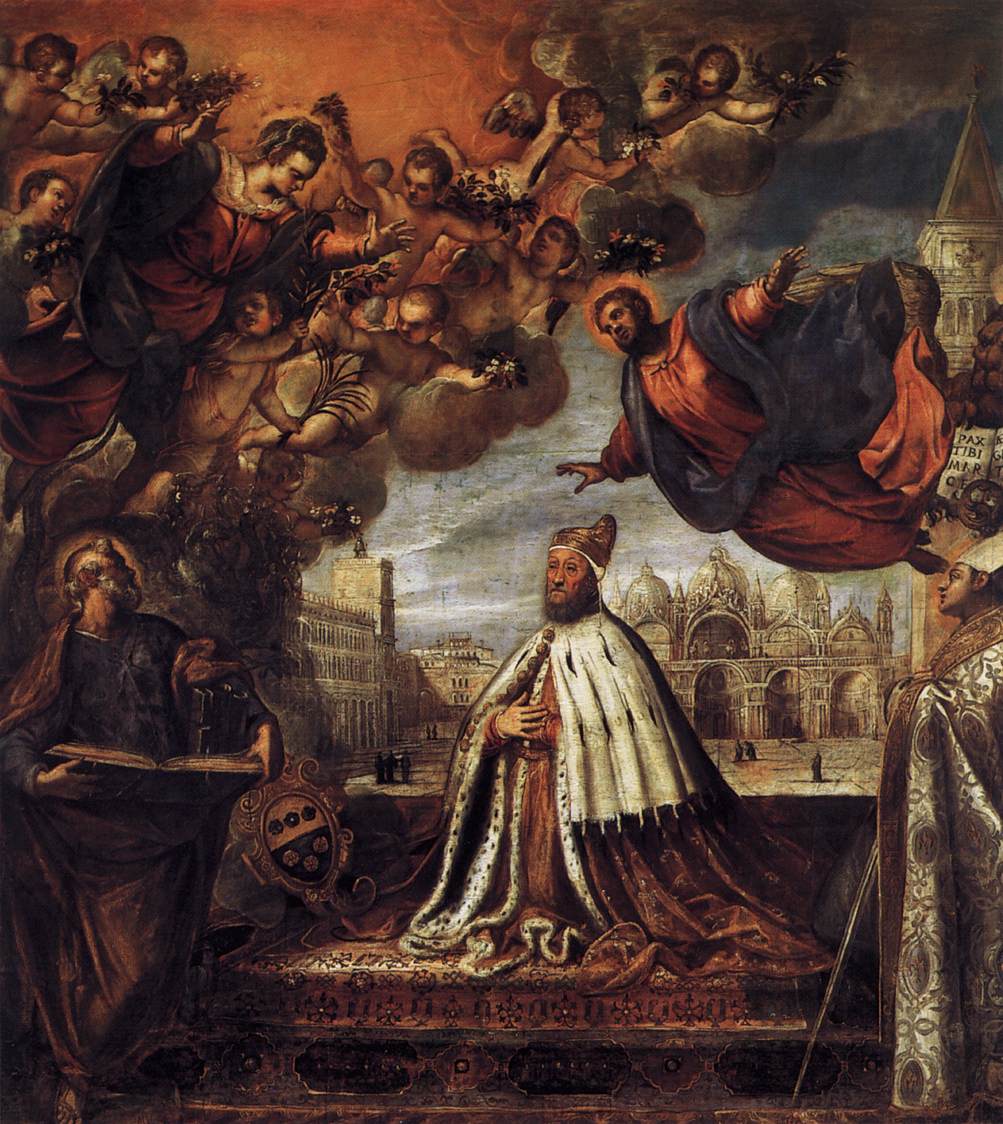The detailed painting appears to be a religious scene, possibly from the Renaissance era, reminiscent of the style seen in the Sistine Chapel. Various figures, including men, women, and children, are depicted floating or flying in the air, dressed in a variety of cloaks and gowns in hues of tan, blue, and orange. Below these celestial figures stands a man who appears kingly or of high religious status, adorned in a regal outfit with a white cape and a tall brown hat. He holds his hands to his chest while standing on a platform. To his right is another prominent figure in a large gown, with a long-sleeved shirt, holding an open book. Behind them, the scene extends to an outdoor backdrop with a cityscape that might suggest Venice, complete with chapels and a royal palace, specifically resembling St. Mark's Square. The sky above is partly visible through the ensemble of floating figures, adding a sense of depth and antiquity to this European painting.